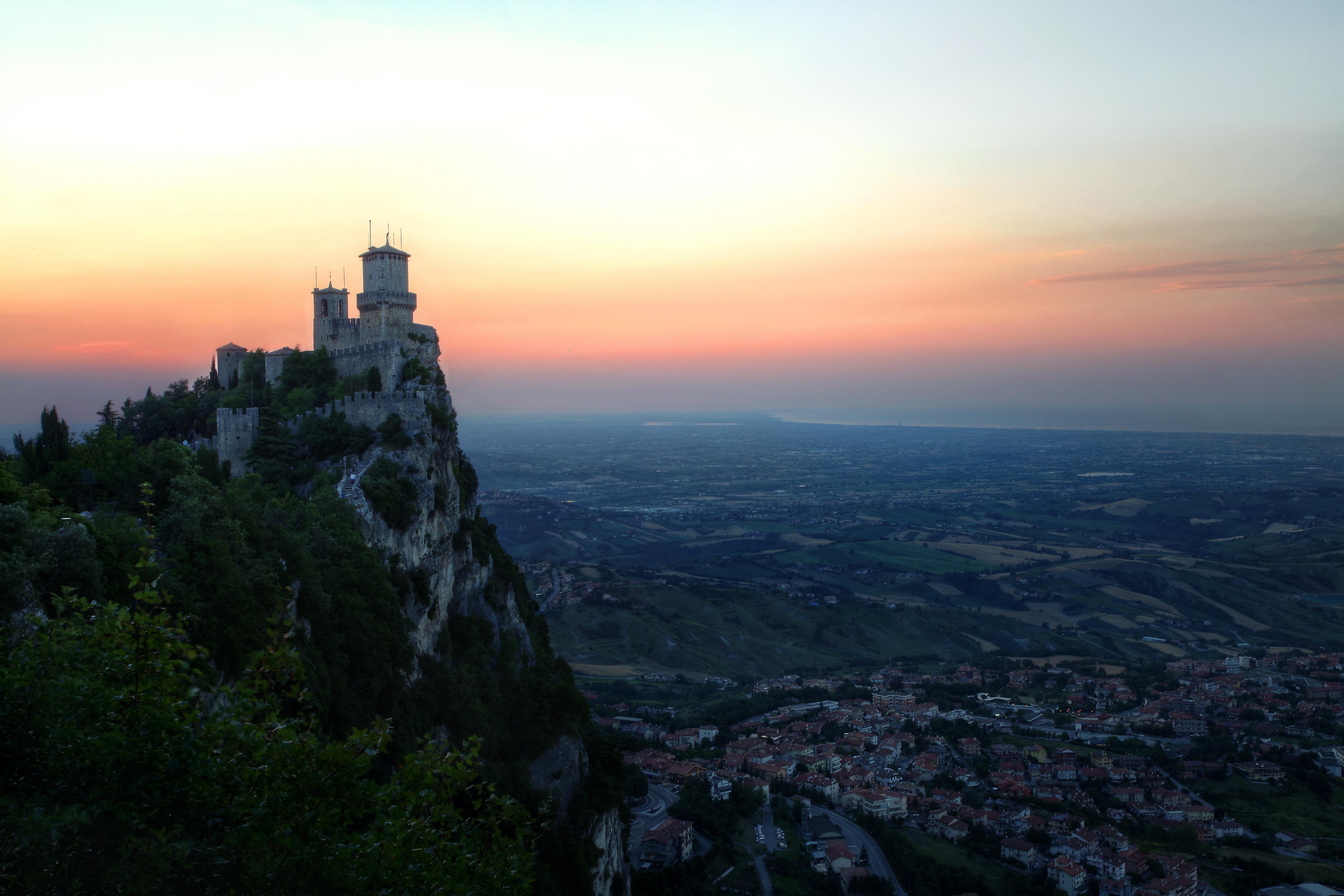The photograph captures the Guaita Tower of San Marino at either sunrise or sunset, perched on a towering cliff on the left side of the image. The fortress appears seamlessly integrated into the rocky outcrop, surrounded by abundant trees and shrubbery. The tower overlooks a vast valley filled with buildings featuring predominantly white walls and terracotta roofs, which are mostly shadowed under the dusky light. The valley below is dotted with lush green fields and distant bodies of water. The sky above transitions from pale blue to pink and orange hues, forming a slightly hazy yet breathtaking backdrop. A distinctive bright yellow arc, indicative of the rising or setting sun, illuminates the scene with soft pink and blue tones, enhancing the serene and majestic atmosphere of this European landscape.